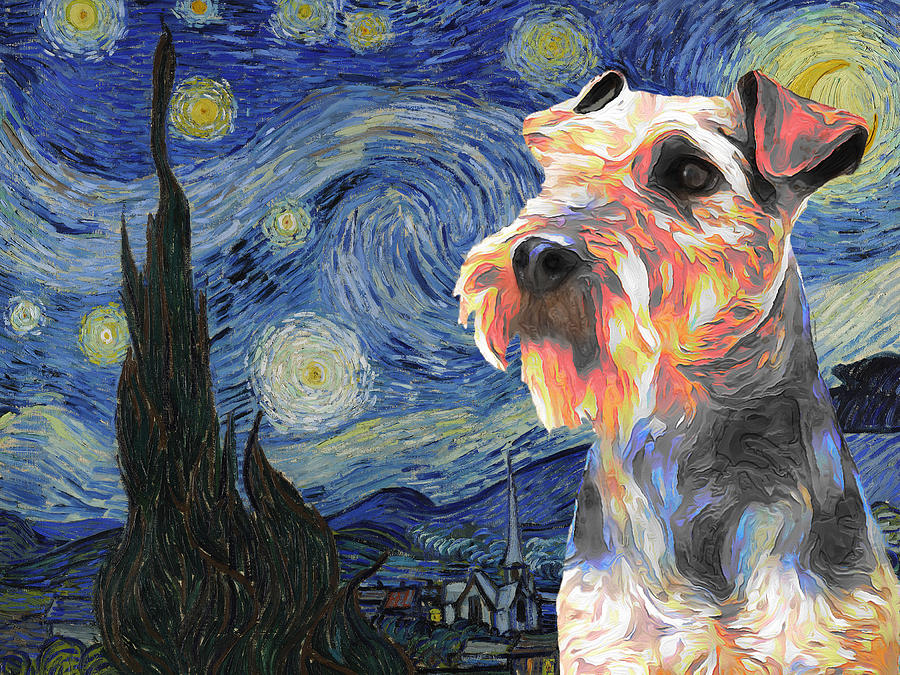The image is a rectangular painting inspired by Vincent van Gogh's "Starry Night." The background features Van Gogh's iconic swirling sky in hues of blue, yellow, and hints of black, punctuated by bright, circular yellow swirls that depict stars. On the left side of the painting, there is a black, swirling structure resembling a cypress tree. In the middle towards the bottom, a small village with distinctive blue rolling hills, a little church, and other small structures can be seen, capturing the tranquil essence of the original masterpiece. However, this version introduces an interesting twist on the right side: a close-up of a schnauzer dog painted in a similar swirling style. The dog, which takes up almost the entire right half of the image, is rendered in shades of white, orange, yellow, dark gray, and red. It stands with its ears pinned back, a black nose, and one visible brown eye, looking off to the left side. This captivating blend of classic art and contemporary creativity brings a charming and unexpected addition to the iconic scene.